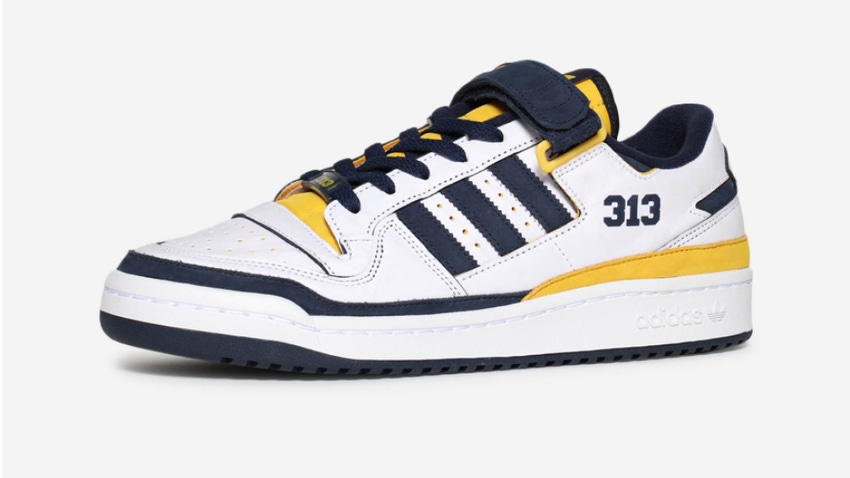This image features a left-side Adidas sneaker set against a white background. The main body of the shoe is primarily white, with navy blue and yellow accents. The navy blue sole transitions into a white midsole, while the toe area casts a dark shadow on the backdrop. The sneaker includes functional navy blue shoelaces and a matching velcro strap for additional support. The tongue and a stripe on the bottom of the sole are both highlighted in vibrant yellow. The number "313" is prominently displayed near the neck of the shoe in blue. Additionally, an "Adidas" label is visible on the base of the shoe. The overall composition of the photograph emphasizes the distinct color palette and design elements of the sneaker while showcasing it prominently in front of a clean, white background.